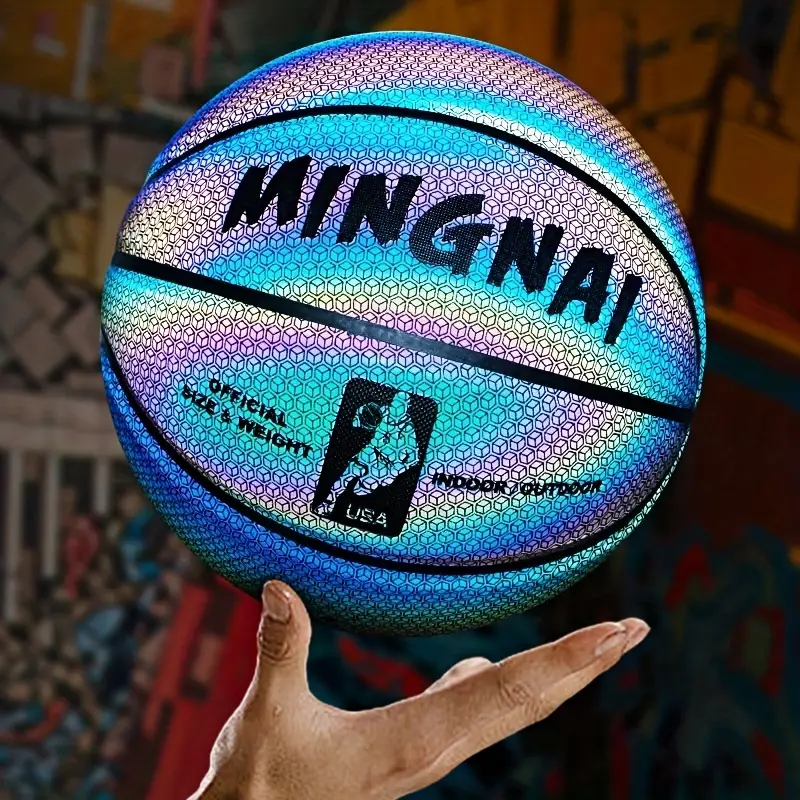In this vibrant and intriguing image, we see a detailed close-up of a unique basketball held by a single outstretched right hand, with only the thumb making contact. The basketball itself is not the traditional brown but instead features brilliant hues of blue, purple, and yellow, with black bands encircling it. The ball is adorned with the text "M-I-N-G-N-A-I" in block-style, oriental-appearing letters, and includes the phrases "official size and weight" on the left and "indoor-outdoor" on the right. Additionally, there’s a silhouette of a basketball player in a running pose holding the ball under their arm, accompanied by the word "USA." The background of the image is a blurred mix of colors, with hints of painted columns or structures adding a layer of depth, contributing to the overall impression that this is a composite of a photograph and a painting. The vibrant colors of the ball, coupled with the subtle, muted backdrop, make it a striking and visually captivating composition.